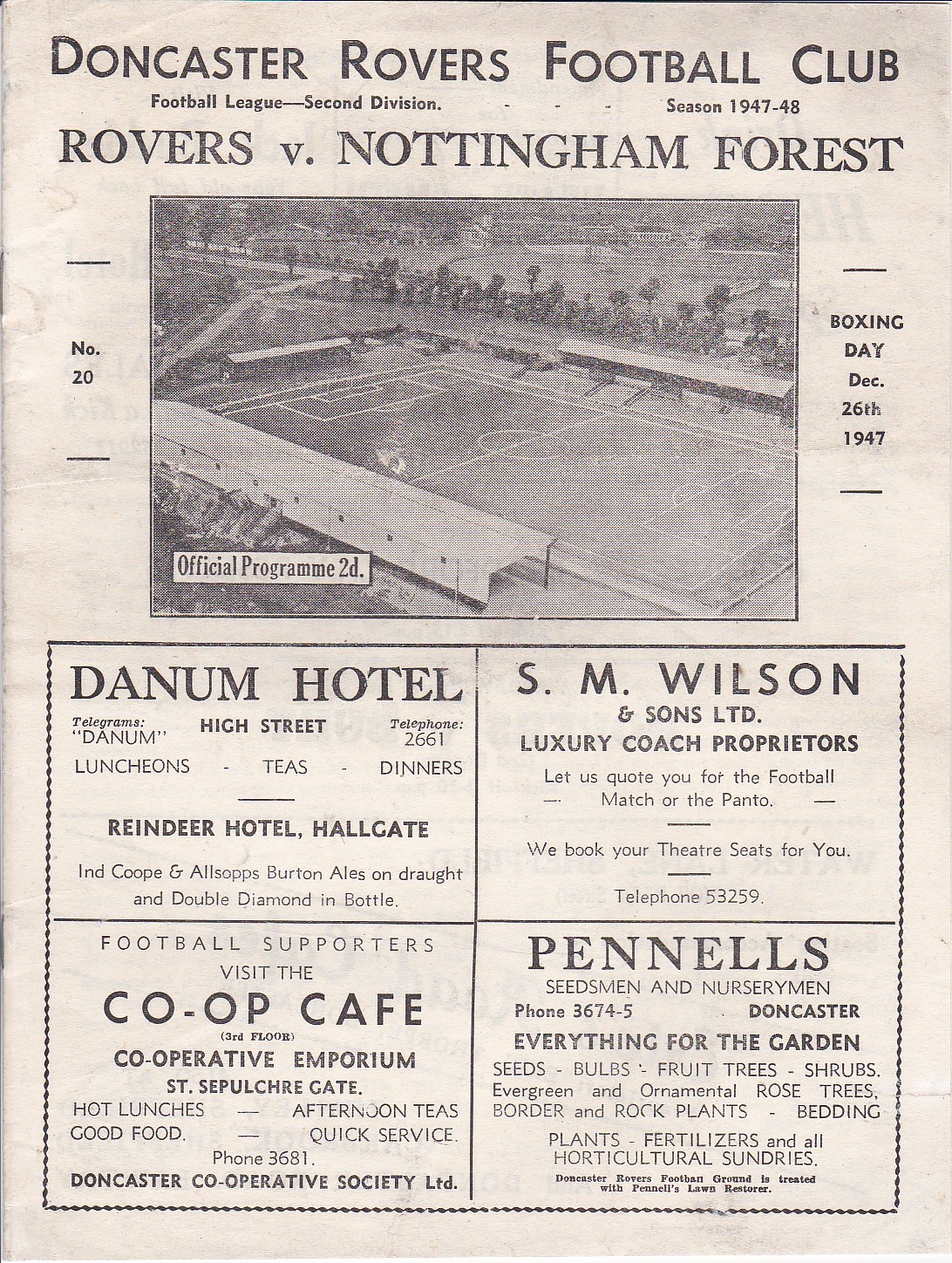This image appears to be an old newspaper article or flyer announcing a notable football match. It features a sepia-toned, black-and-white photograph of an aerial view of a soccer field, surrounded by trees, with some blurry details in the background. Across the top in bold, black letters, it reads "Doncaster Rovers Football Club, Football League, Second Division, Season 1947-48." Below this header, it prominently displays "Rovers versus Nottingham Forest." To the left of the photo, there is "Number 20," while the right side notes "Boxing Day, December 26, 1947." Below the image is a section with four advertisements arranged in a rectangular box: the top left is for Danham Hotel, the top right for S.M. Wilson & Sons Ltd. (Luxury Coach Proprietors), the bottom left for Co-op Café (highlighting offerings like hot lunches, good food, afternoon teas, and quick service), and the bottom right for Pennell's Seedsmen & Nurserymen. The text is accompanied by the words "Official Programme," although spelled uniquely. This detailed caption encapsulates the nostalgic and historical value of the event from the era.